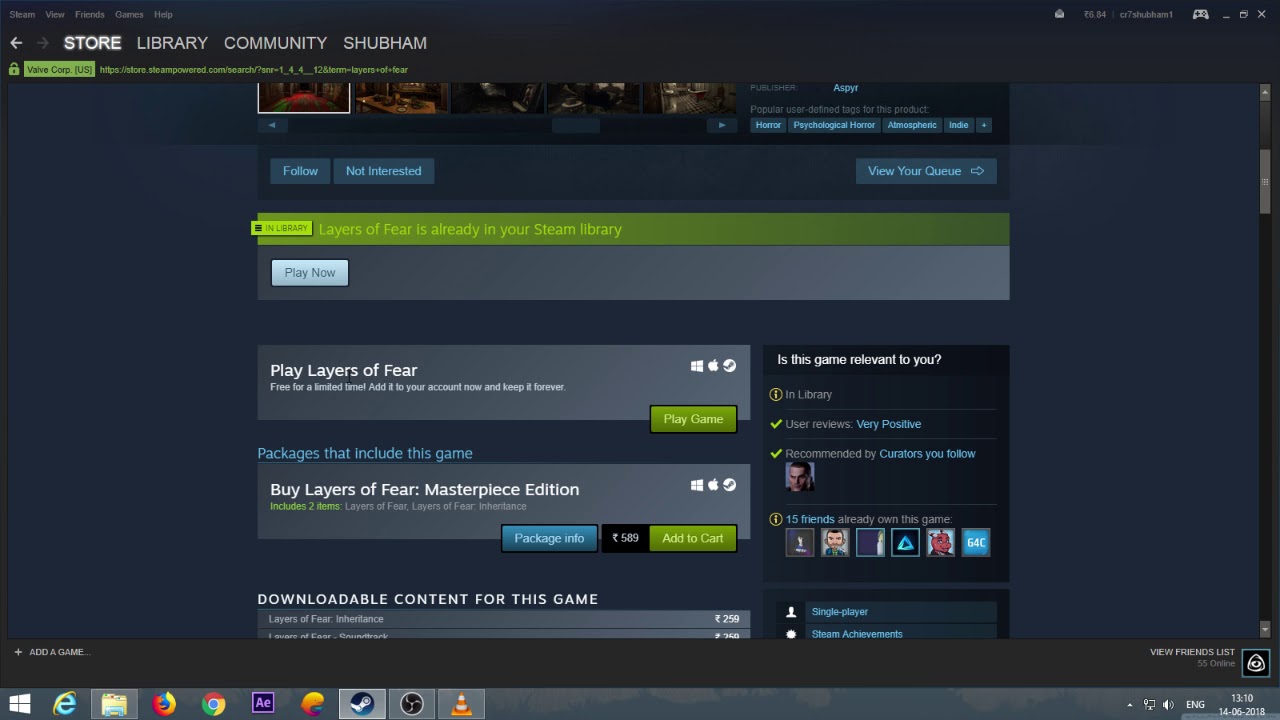This is a screenshot of the Steam platform, featuring a dark-themed interface with blue and green highlights. At the top of the screen, a menu bar displays options labeled Store, Library, Community, and Shubham. The Store tab is currently selected, indicating that the user is browsing the Steam Store page. Prominently displayed at the top are game images and promotional content.

The highlighted section of the page announces that the game "Layers of Fear" is already in the user's Steam library, accompanied by a green "Play Now" button. Below this, it offers additional options such as "Play Layers of Fear," "Buy Layers of Fear Masterpiece Edition," and other downloadable content for the game.

To the left, a sidebar contains various polls and links, adding interactive elements and quick navigation options for the user. The combination of dark colors and vibrant highlights makes for a visually striking and easily navigable interface, consistent with Steam's signature style.